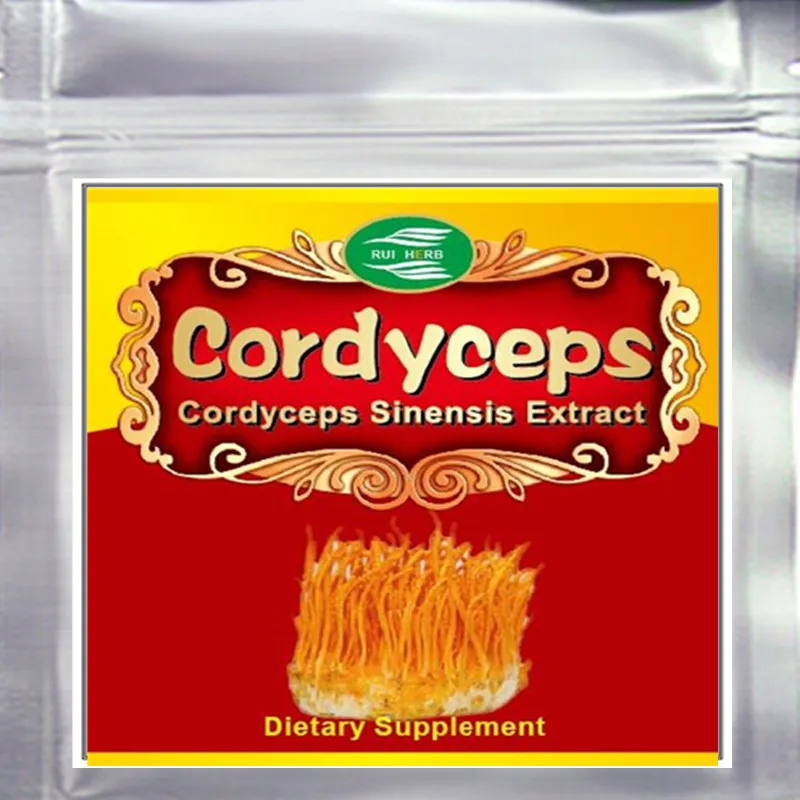The image is a square, six-inch by six-inch, close-up of a silver foil package labeled "Cordyceps Sinensis Extract". The top part of the packaging features finger notches and a tearable top, which can be resealed via a zip-lock strip below. A central square label dominates the package, outlined by a white border with thin gray stripes inside. This label has a yellow background at the top, transitioning to red at the bottom, with an additional thin yellow stripe along the bottom edge.

At the very top center of the label, there's a green oval logo with red text that reads "RUI HERB." Directly beneath, in gold letters on a red background, is the product name "Cordyceps," followed by "Cordyceps Sinensis Extract" below it. The bottom section of the label features an image of the cordyceps fungi, depicted as yellowish-orange, hair-like structures standing up against the red background. At the very bottom, in bold yellow letters, are the words "Dietary Supplement."